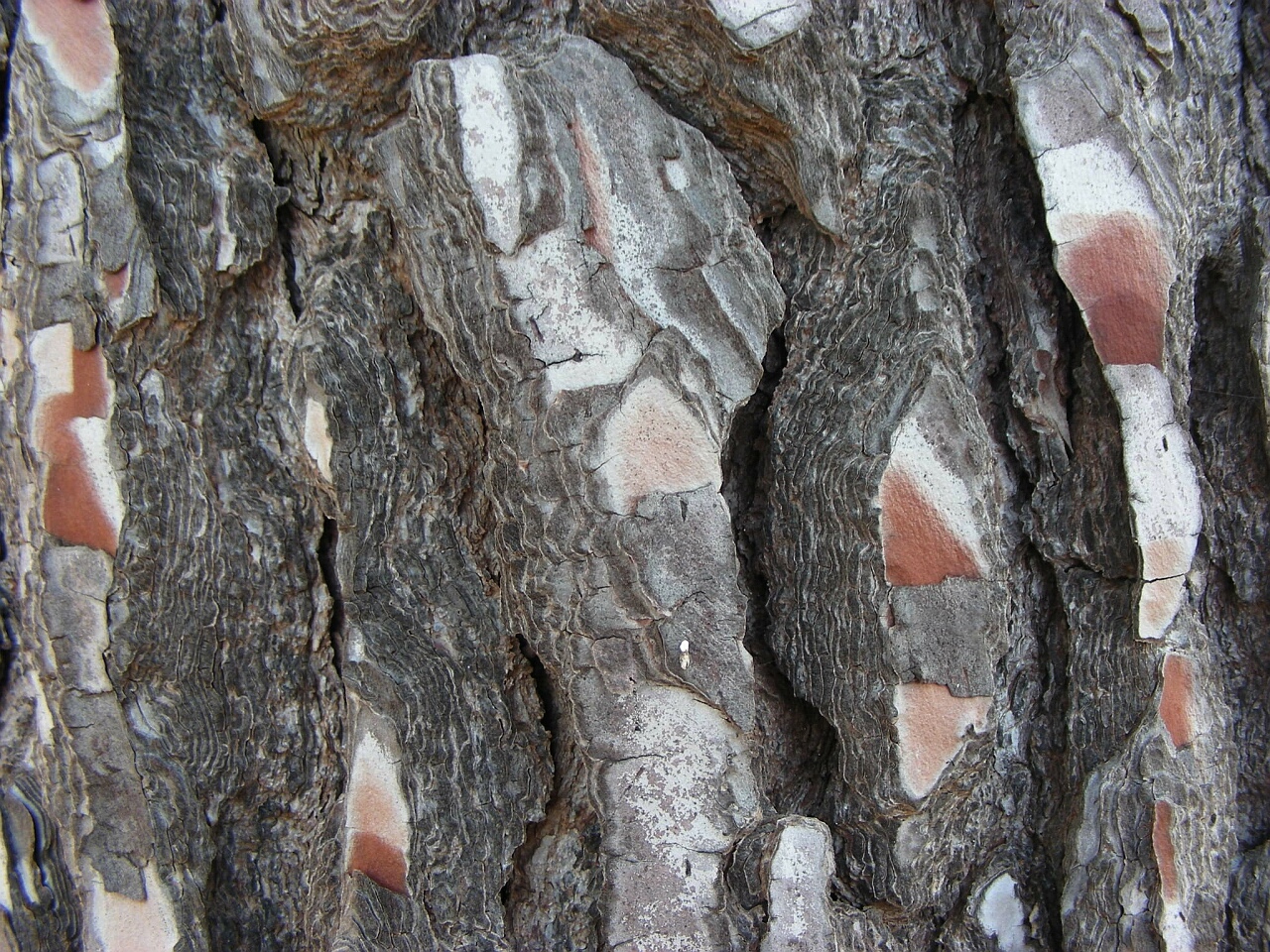This close-up photograph appears to be taken outdoors and showcases a textured surface that mimics the appearance of tree bark. The dominant hues are various shades of gray, interspersed with touches of brown and white. The surface features a rough texture with vertical striations, suggesting a north-south orientation typical of tree bark. However, the image could also be interpreted as an abstract artwork or even stones viewed from an unusual angle. Despite this ambiguity, the prevalent grayish tones and the vertically aligned texture are the most distinguishing characteristics.